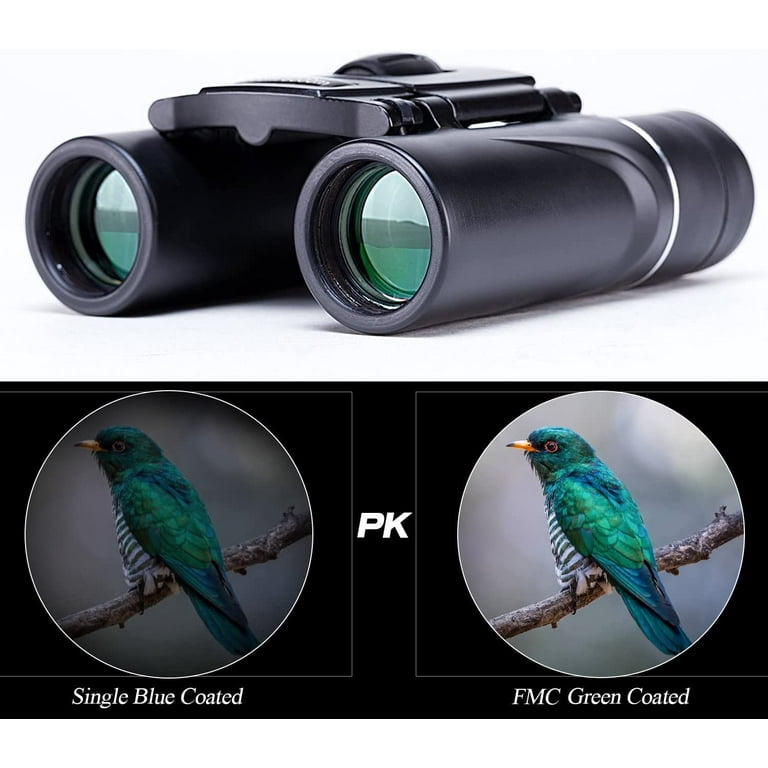This advertisement showcases a pair of black PK birdwatching binoculars, highlighted against a stark white background. The photorealistic image at the top reveals the binoculars' detailed design: two elongated spherical cases connected by a top square piece, with green-tinted lenses. Below this is a horizontally split comparison of two images displaying the view through different coatings of binocular lenses. Both images feature a vibrant green and blue bird with a black and white striped body perched on a branch. The left half, labeled "single blue coated," shows a darker, hazier view, while the right half, labeled "FMC green coated," presents a clearer, sharper, and more brilliant image. The central placement of "PK" emphasizes the brand, illustrating the binoculars' superior visual quality with the FMC green-coated lenses.